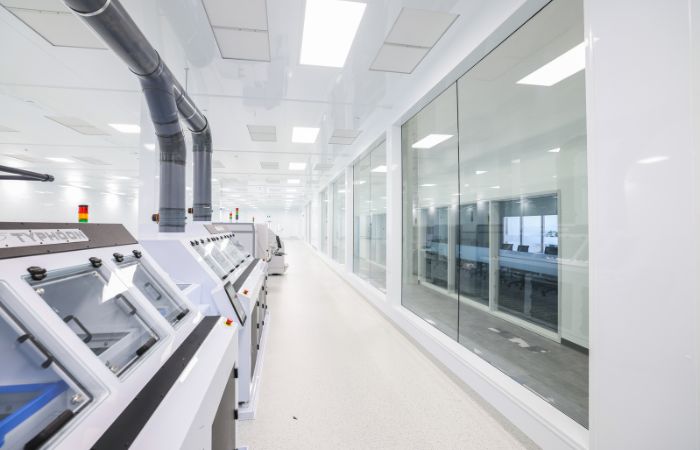The photograph depicts a bright, well-lit laboratory or facility with highly reflective, white floors and ceilings, which mirror the surrounding environment. On the left side, there is a line of several different white machines featuring small glass windows and doors with dark handles. These machines have gray tops and are equipped with green, yellow, and red lights. The prominently labeled "Typhoon" machine is situated at the far left. Adjacent to it, the second machine features large black pipes extending upwards and connecting to other pipes running along the ceiling. On the right side of the image, there is a long stretch of clear, floor-to-ceiling windows providing a view into another area with a gray walkway and an additional white wall primarily composed of large windows. The ceiling of the room is fitted with long rectangular lights that stretch into the distance, enhancing the bright and sterile ambiance of the facility.